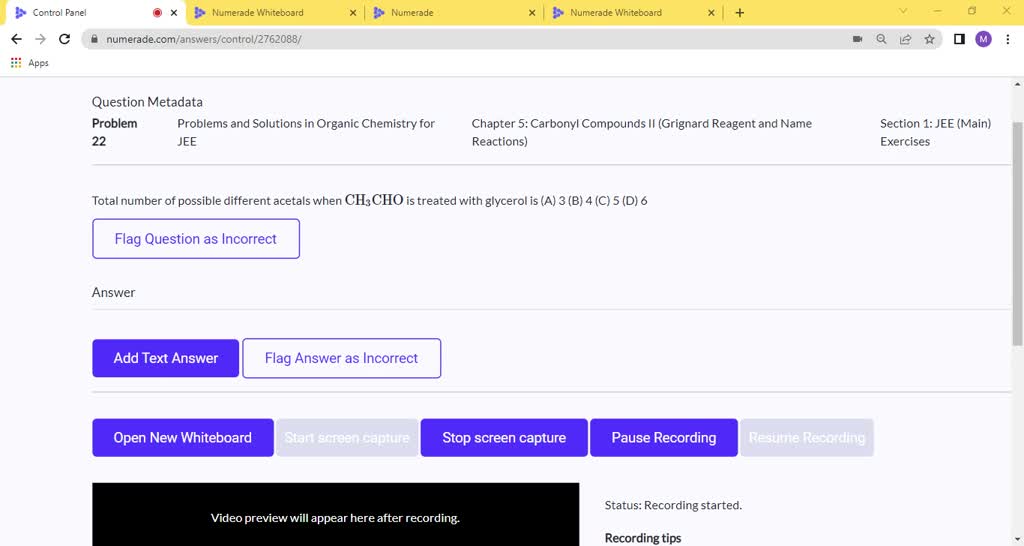The image is a screenshot from a website, featuring a predominantly white backdrop. Along the top, there's a yellow bar spanning the width of the page. In the upper left corner, there's a small white tab labeled "Control Panel" in black text, marked by a purple Play logo at a sideways angle. Adjacent to it is a red circle with a black 'X' for closing. Next is another purple Play logo, followed by "Enumerate Whiteboard" in black text, and another black 'X'. This pattern repeats with minor variations.

On the right end of the yellow bar, there are icons in black: a drop-down logo, a minus, a box, and an 'X'. Below this, the toolbar displays navigation arrows, a refresh icon, and a search bar containing the URL: "Enumerate.com/answers/control/2762088/".

Directly below, there is a multicolored 3x3 dot square icon labeled "Apps". Beneath this, it reads "Question Metadata", "Problem", and "22". Next to "Problem", it states "Problems and Solutions in Organic Chemistry, 4" followed by "JEE", "Chapter 5, Carbonyl Compounds", and "(Grignard, Regenerate, and Name Reactions)". To the right, it notes "Section 1, JEE (Main)".

Below this heading, the main body showcases a problem statement: "Total Number of Possible Different Acetyls when CH3CHO is treated with Glycerol." Options are labeled: "(A) 3", "(B) 4", "(C) 5", and "(D) 6".

There are interactive buttons for user actions:
- A white box with a purple outline labeled "Flag Question as Incorrect"
- A black label "Answer"
- A blue box with "Add Text Answer" in white
- A white box with a blue outline labeled "Flag Answer as Incorrect"
- A blue box with "Open New Whiteboard" in white
- A gray box labeled "Start Screen Capture" in white
- A blue box with "Stop Screen Capture" in white
- A blue box with "Pause Recording" in white
- A gray box with "Resume Recording" in white

At the bottom, a black box states "Video Preview will appear here after recording," with "Status: Recording Started." Subtext reads "Recording Tips".